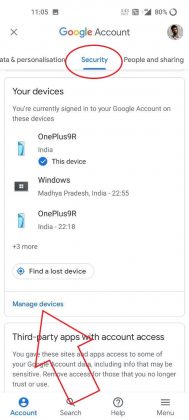Here's a refined and detailed caption:

---

This image depicts a smartphone screenshot with an all-white background. At the top left corner, the time is displayed as 11:05. On the opposite corner, the battery life is shown at 80%, alongside some gray status icons. Centrally aligned, a heading reading "Google Account" is prominently displayed. To its left, there is a gray 'X' icon, and to its right, a profile picture of a man.

Just below this heading, three menu options are listed: "Data & Personalization," "Security," and "People & Sharing". The "Security" option is highlighted in blue and encircled with a red circle. Moving down, a section titled "Your devices" notes that the user is currently signed into their Google account on several devices.

Details of the devices include:
1. **OnePlus 9R (India)** - Marked with a blue check mark and labeled as "This device".
2. **Windows (India)** - Listed with the time 22:55.
3. **Another OnePlus 9R (India)** - Listed with the time 22:18.
4. A line stating "+3 more".

Further down, there are options labeled "Find lost device" and "Manage devices" in blue. Another section named "Third-party apps with account access" appears next. This section elaborates that certain sites and apps have access to the user's Google account data, including potentially sensitive information. A prompt indicates the possibility of revoking access for those no longer deemed trustworthy.

At the bottom of the screen, there are four icons: an "Account" button, a "Search" button, a "Help" button, and a "Hamburger" menu icon.